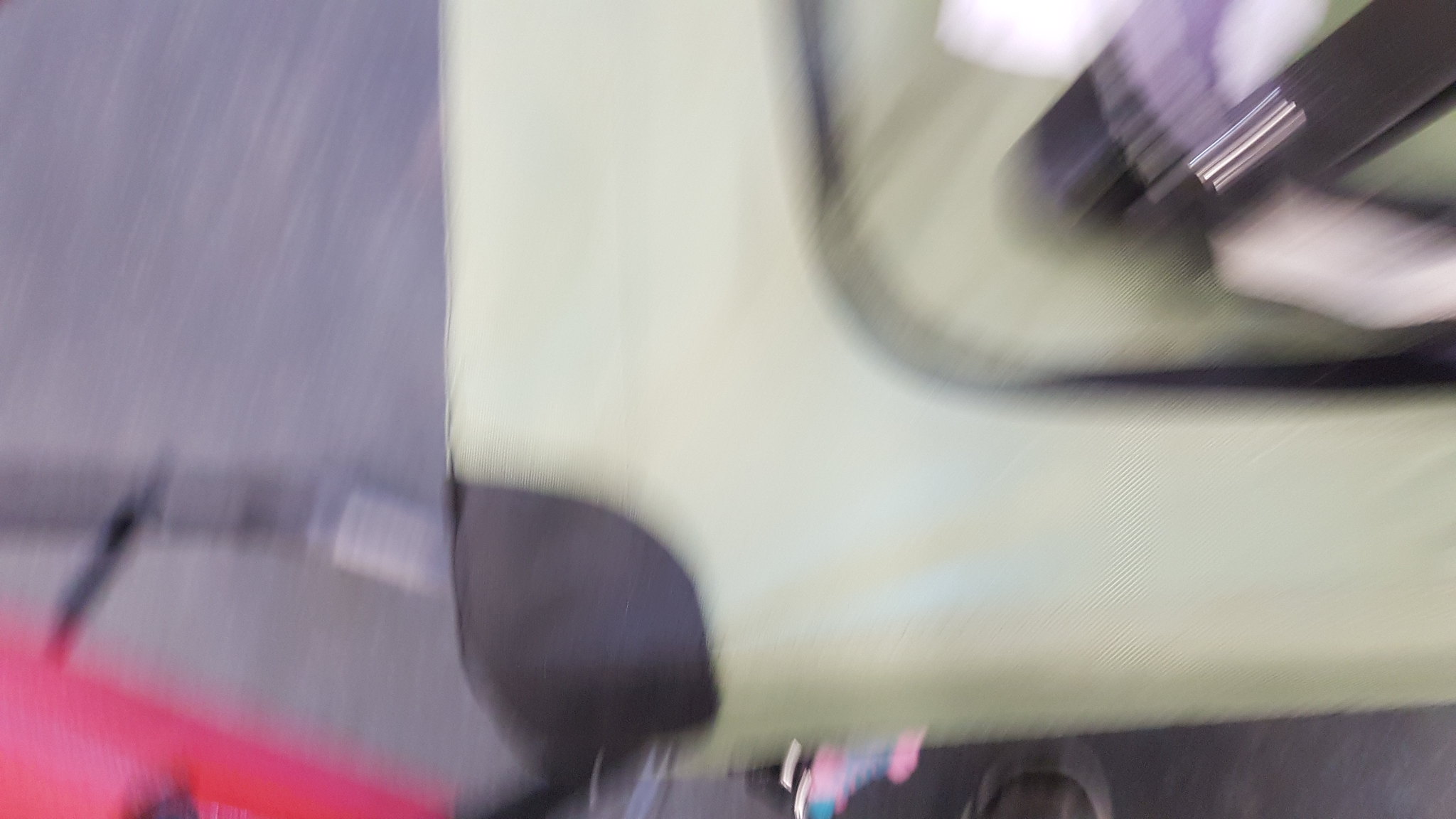This image captures the bottom left corner of a rounded table covered in green felt. A distinct black cutout is visible at the corner, suggesting a possibly functional or decorative feature. The table is positioned above a gravel-covered surface, with a faint hint of red visible in the background, though its nature remains unclear.